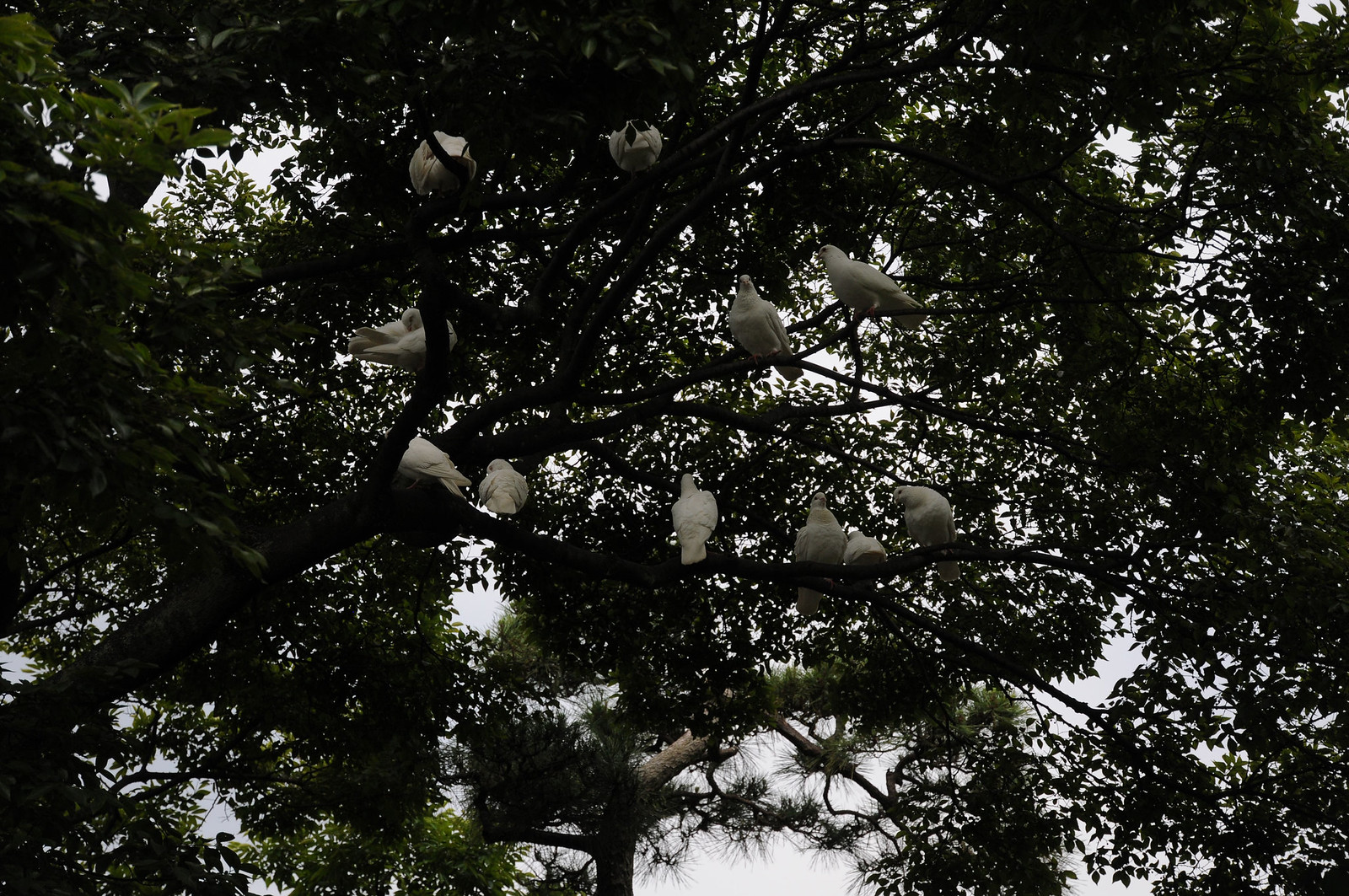In the photo, an upward perspective captures a tree with dense, dark-leaved branches juxtaposed against a gray sky, creating a dramatic contrast. Around 11 white doves are perched on various branches, their bright feathers standing out starkly against the predominantly black and dark green hues of the tree. The sky appears either cloudy or indicative of early evening or dawn, adding to the overall dim lighting and shadowy ambiance of the scene. Despite the poor lighting, the doves are prominently visible, perched serenely amidst the thick, dark foliage that dominates approximately 95% of the image.